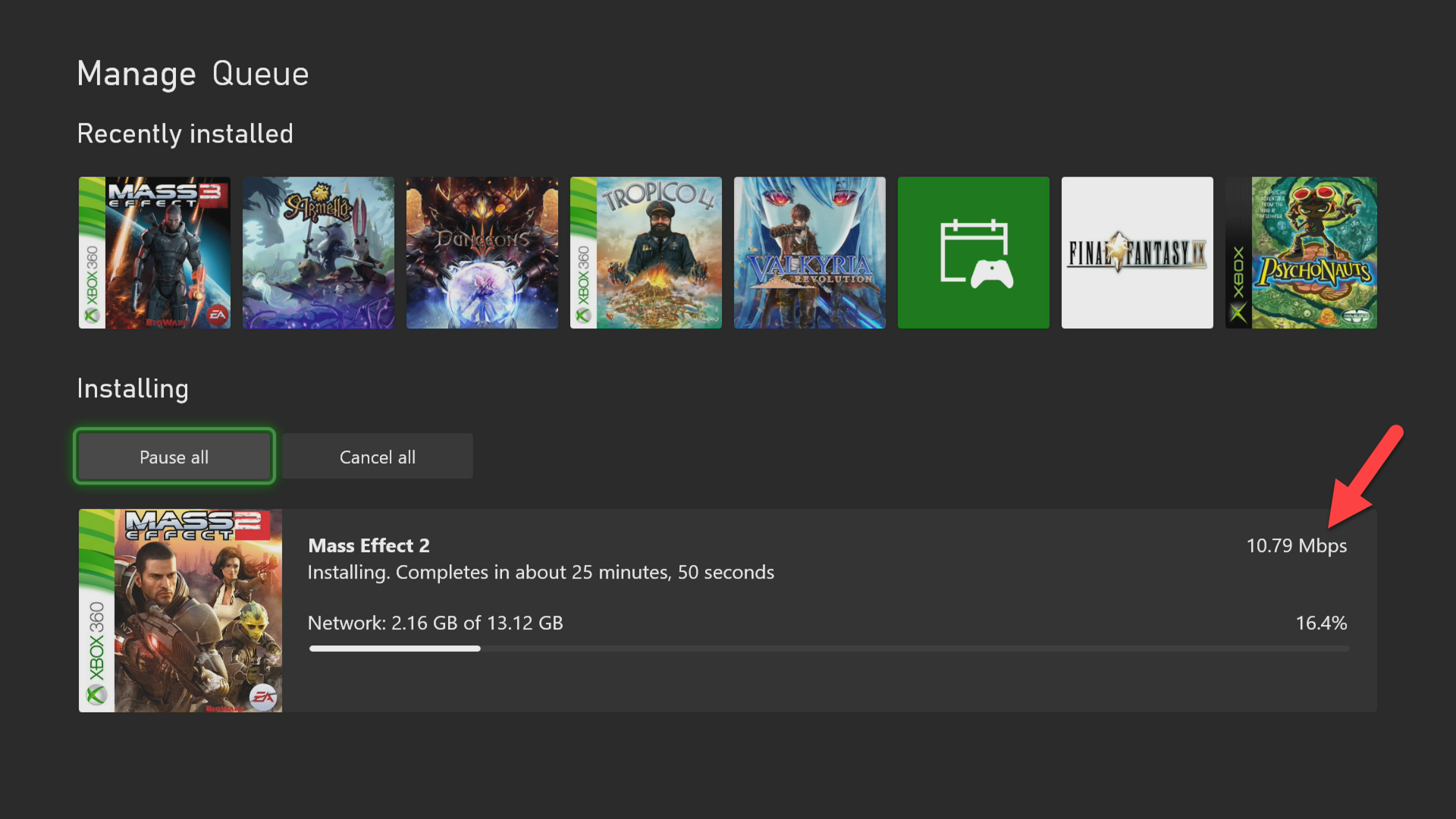The image, sourced from a website recently displaying the installation of Manage Q, showcases an array of video game covers with vivid detail. Prominently featured is the cover for "Mass Effect 3" for the Xbox 360, depicting a heavily armored character. Alongside it, we see the cover of "Tropico 4," with a suave man dressed in a captain's suit, set against a dramatic backdrop of an island and raging fire. Adjacent to these is the striking cover of "Valkyria Revolution," highlighting a blue-haired, red-eyed anime-style character. Among the collection, the classic "Final Fantasy" cover stands out, as well as the quirky and imaginative game, "Psychonauts." The compilation provides a rich visual feast for gaming enthusiasts, blending elements of sci-fi, strategy, role-playing, and adventure genres.